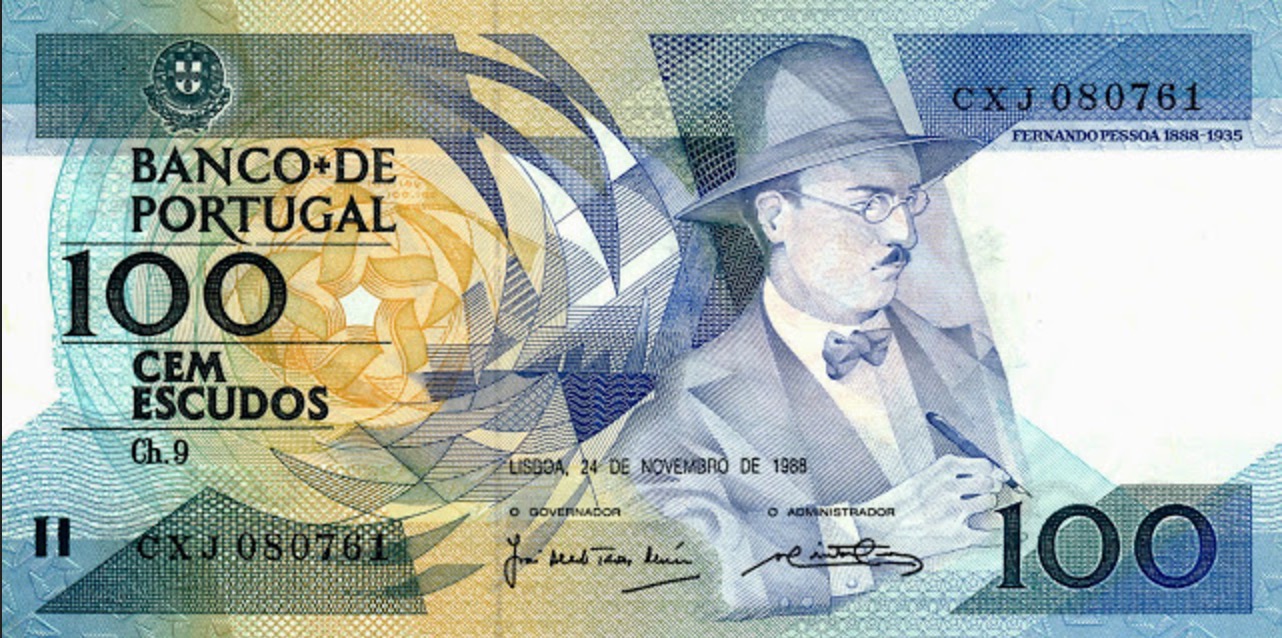This image features a 100 Escudos banknote from Portugal, prominently displaying a multi-colored design that transitions through shades of blue, teal, turquoise, yellow, and green, with a geometric and pointillist overlay primarily in navy blue. The banknote is inscribed with "Banco de Portugal" at the top left, followed by "CEM ESCUDOS" and the number "108." Below that, the phrase "Chapter Nine" appears along with the serial number "CXJ080761," which also repeats at the bottom left next to two vertical lines. The banknote features a portrait of Fernando Pessoa on the right side, identified by the years "1888-1935" beside him. Pessoa is depicted wearing a hat, glasses, a bow tie, and holding a pen in his right hand, positioned above the number "100." The bill also bears the signatures of the Governor and the Administrator in the right section. The overall background features a detailed pattern combining a spiral design on the left third and Fernando Pessoa on the right third, set against a backdrop that integrates white areas within the intricate colorful pattern.